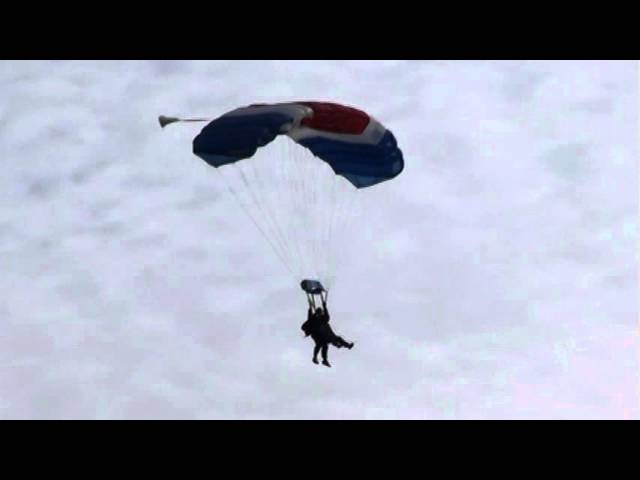The image captures a striking silhouette of two individuals parachuting, centered against a moody, overcast sky filled with varying shades of gray and blue clouds. Both figures hang suspended from the ropes of a parachute that features a distinctive color pattern: red at its core, flanked by a white stripe, and blue on either side. The front person has their legs extended forward, while the person in the back has their legs hanging down and arms raised, likely gripping the parachute ropes. The overall lighting casts the figures in near-total silhouette, enhancing the dramatic contrast with the slightly better-lit parachute. The photograph is framed with thin black bands along the top and bottom, encompassing a predominantly blue, black, and gray palette, against which the parachute's vibrant colors stand out starkly, adding a dynamic element to the otherwise subdued background.